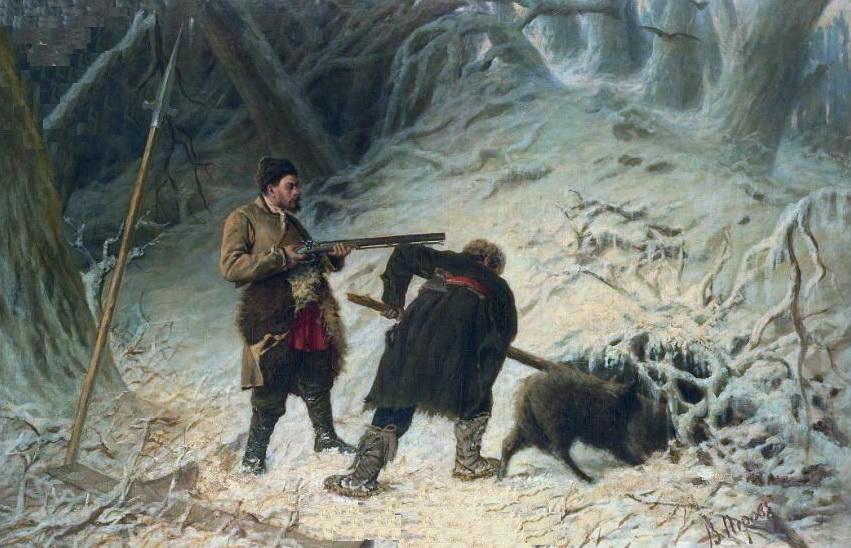This evocative winter scene painting portrays two men hunting in a snow-covered forest as dusk falls. The men, clad in warm clothing including boots, long coats, and possibly fur hats, are positioned near the entrance of a burrow. One man stands ready with a double-barrel shotgun, while the other is crouched, poking a long stick into the hole. A dog, its tail between its legs, burrows into the hole ahead of them. Nearby, a large spear with a silver tip stands upright, adding to the sense of readiness and tension. The surroundings are marked by the shadows of tall trees and a log resting over the burrow's entrance, contributing to the scene's overall sense of quiet anticipation.